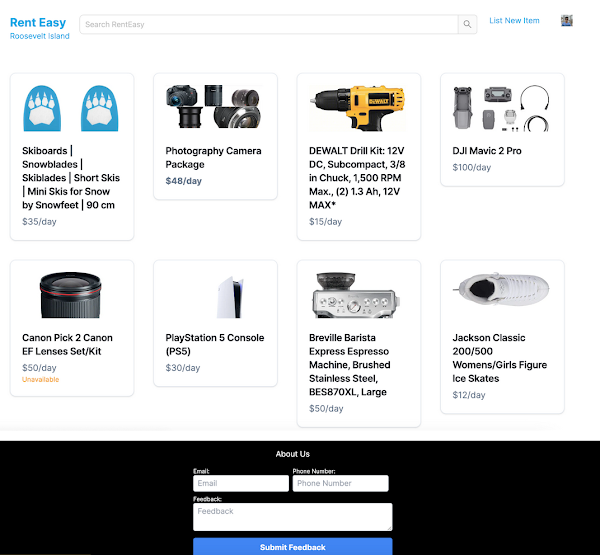The image is a horizontally rectangular screen capture from a rental website with a predominantly white background. In the upper left corner, the website's name "Rent Easy Roosevelt Island" is displayed in blue. To the right of this, there is an elongated search field, followed by a "List New Item" button.

Below, the page is organized into two rows, each containing four listings, all neatly enclosed in light gray borders. The items and their rental details are as follows:

**First Row:**
1. Ski Boards, Snow Blades, Ski Blades, Short Skis, Mini Skis for Snow (by Snow Feet), 90 centimeters - **$35 per day**.
2. Photography Camera Package - **$48 per day**.
3. DeWalt Drill Kit, 12 Volt DC, Subcompact 3/8 Inch Chuck, 1500 RPM Max - **$15 per day**.
4. DJI Mavic 2 Pro Drone - **$100 per day**.

**Second Row:**
1. Canon PIC 2 Canon EF Lenses Set Kit - **$50 per day** (listed as unavailable).
2. PlayStation 5 Console - **$30 per day**.
3. Breville Barista Espresso Machine - **$50 per day**.
4. Jackson Classic 200-500 Women’s/Girls’ Figure Ice Skates - **$12 per day**.

Each listing includes the item's name, a brief description, and the corresponding daily rental rate, providing potential renters with concise information.